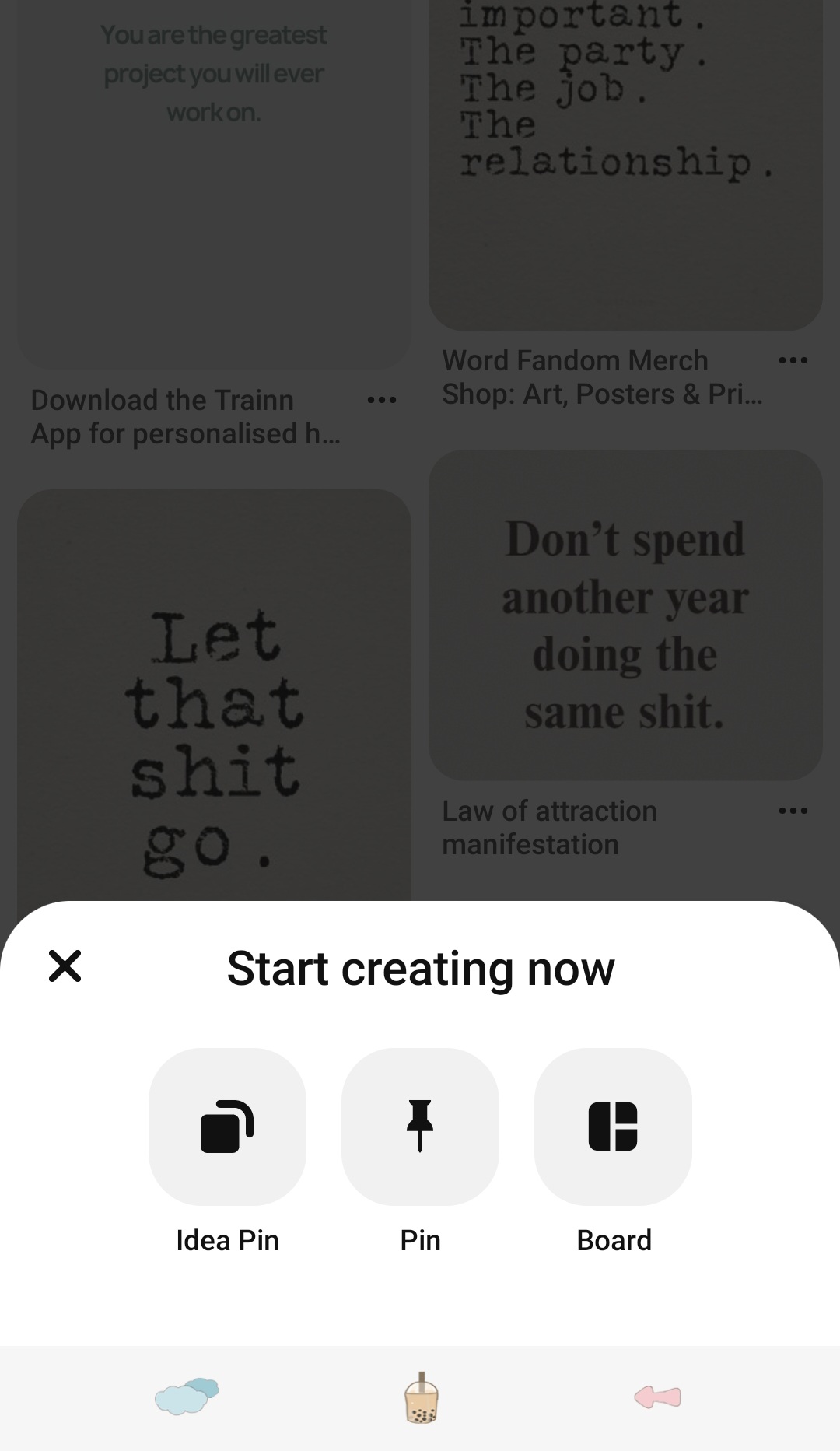The image appears to be a screenshot from the Pinterest platform, showcasing a mixture of motivational quotes and prompts for content creation. The background displays four typical motivational sayings that one might encounter on social media, specifically Pinterest. These sayings are grayed out and read as follows: "Don't spend another year doing the same shit," "Let that shit go," "Everything important—the party, the job, the relationship," and "You are the greatest project you will ever work on." 

Overlaying this background is a stark white pop-up box that prominently reads "Start Creating Now." Within this box, there are phrases such as "Idea Pin," "Pin," and "Board," suggesting a call to action for users to engage with Pinterest's content creation tools. Below these texts, there are icons depicting two clouds, a bucket, and a backward-facing arrow, potentially representing different functions or categories within the app.

The color palette in the image includes blue, brown, pink, black, and gray. Additionally, terms like "Law of Attraction," "Manifestation," "Word Fandom," "Merch Shop," "Art Posters," and "The Train App for personalized" are scattered throughout, hinting at a variety of interests and themes available on the platform.